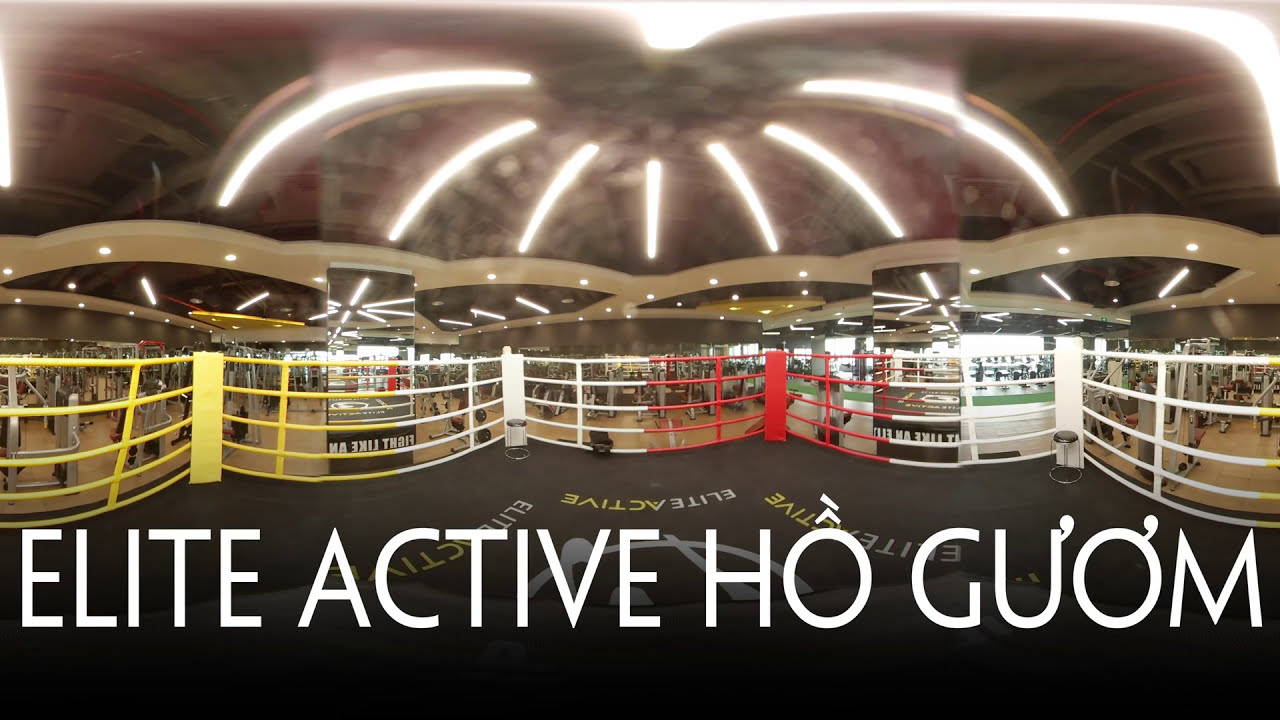This panoramic image captures a vibrant gym setting prominently branded with the name "Elite Active Ho-Guam" in bold, uppercase white font. The gym features a raised area with a distinctive yellow, white, and red guardrail that stretches across the black-floored platform. The flooring itself is adorned with the words “Elite Active” repeated in white and yellow font. The gym is equipped with a multitude of exercise machines, predominantly white, and illuminated by large, arched white lights from the ceiling, which also has an architectural design featuring multiple arches and rounded areas with additional lighting. Although the image is slightly distorted due to its panoramic nature, making it challenging to discern, there appear to be a few people working out amidst the extensive gym equipment. This dynamic setup and the prominent branding suggest that the gym offers a comprehensive environment for fitness and training activities, possibly including specialized areas for boxing or MMA training.